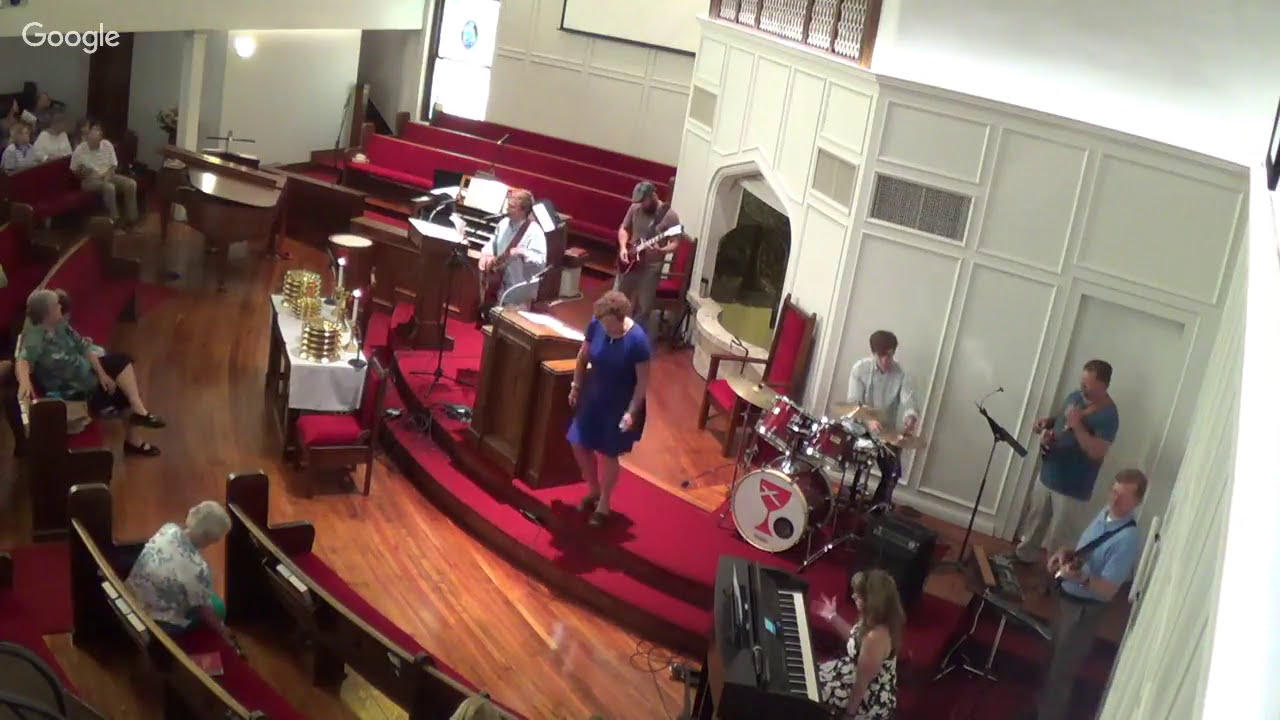The image captures an elevated view of the inside of a church during a musical performance. The stage, designed in a semi-circular shape, is elevated by two steps that are covered in red carpet. The stage and the floor both feature wood paneling, but the edges of the stage remain carpeted. A white wall serves as the backdrop, with doors and glass windows visible.

On stage, a band is performing. Toward the center back of the stage, a person wearing a hat is seen playing the guitar. To their left, another musician in a white shirt also has a guitar and is singing into a microphone. Towards the right side of the stage, a person in a long-sleeved white shirt with dark hair is playing the drums, and another person in a gray t-shirt is standing by them, playing a guitar.

In the front right corner, there is a female performer in a blue gown, holding a microphone, who appears to be the main singer. Additionally, there is another guitarist and a girl sitting at a piano. 

The audience, visible at the left edge of the image, sits on pews arranged in a circular pattern and facing the stage. The pews feature red upholstery and are occupied by various attendees, mostly elderly men and women. A blue-shirted individual can be seen walking down the two red-carpeted steps of the stage. The top-left corner of the image bears a Google watermark.